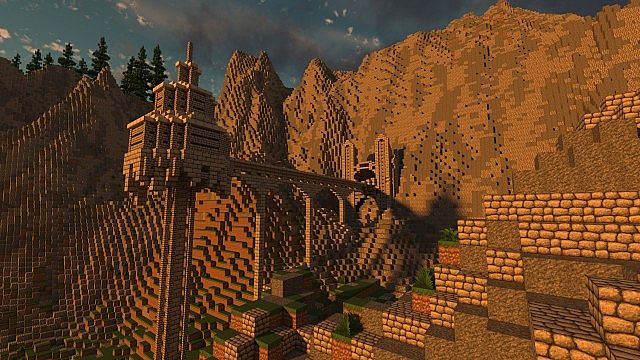The image depicts an intricate and detailed digital artwork, reminiscent of a scene from a video game constructed with a block-like design akin to Minecraft or Lego. Dominating the background is a striking blue sky, imbued with various shades, ranging from a somewhat dark tone to a tail blue hue, interspersed with scattered white clouds. In the top left corner, tall, pine-like trees, resembling Christmas trees, jut out from a jagged brown cliff, enhancing the natural beauty of the landscape. The mountainous terrain stretches across the image, showcasing a mix of dark brown, reddish-brown, and tan hues that resemble layers of brick or Lego blocks.

Centrally located yet slightly shifted to the left, stands a distinctive multi-tiered building, reminiscent of Asian architecture, similar to a wedding cake with small, medium, and larger tiers. This structure appears connected to a wall or bridge extending towards the front and side of the image. On the right side, a terraced landscape of varying geological features, including rock and soil, is visible. The scene also includes green plant life interspersed throughout, and steps that seem to lead up to another area, adding to the complexity and depth of the artwork.